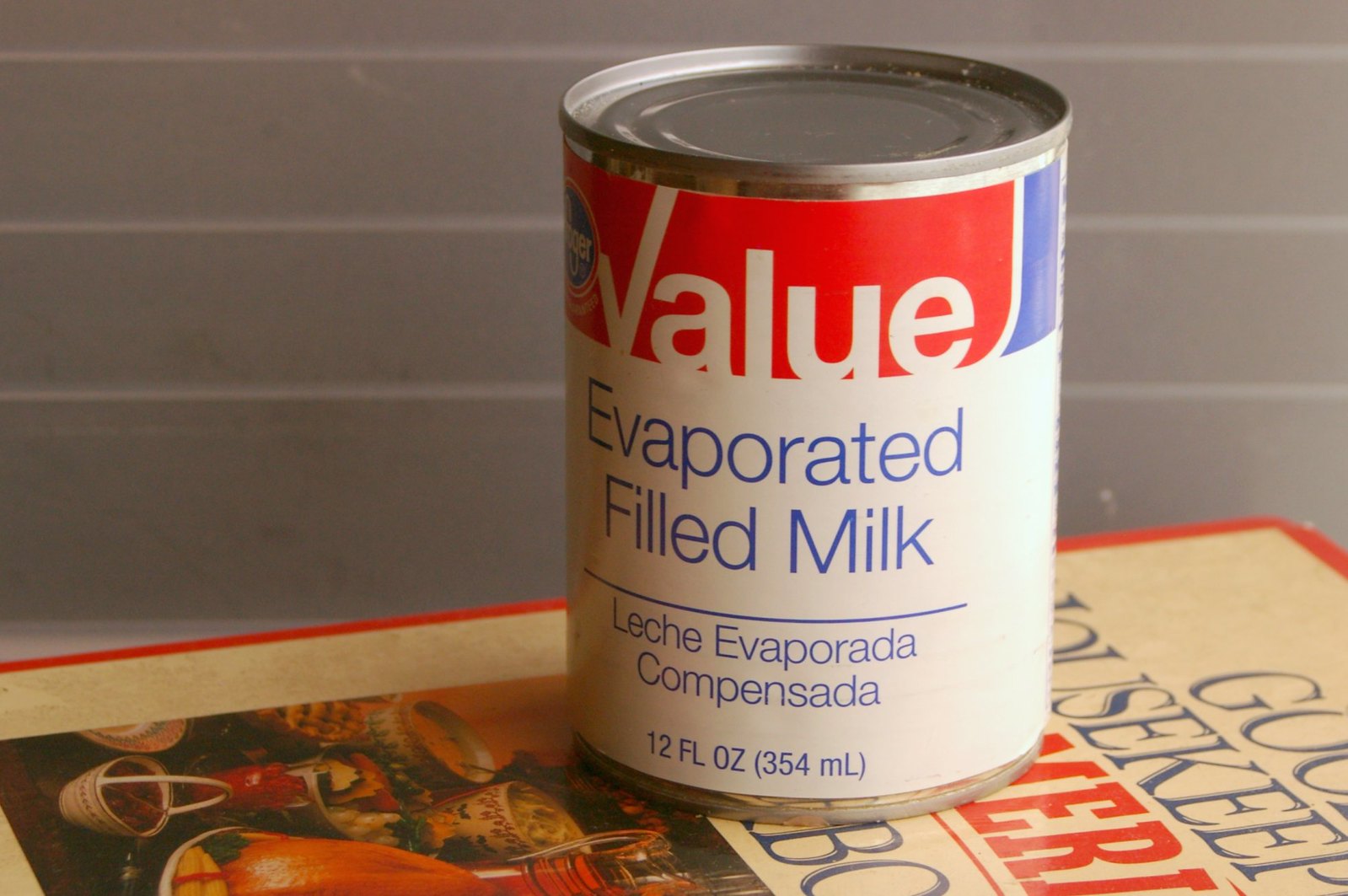The photograph captures a nostalgic and vintage scene. The background features a medium gray wall adorned with subtle white horizontal pinstripes. Seated on a countertop is a well-worn "Good Housekeeping" cookbook with a distinctive reddish-orange spine and a white cover. The title "Good Housekeeping" is prominently displayed, though partially obscured. A faded food photograph embellishes the lower section of the cookbook cover.

In the foreground of this scene, a metal can commands attention. To the left of the can, though not entirely legible, the label may indicate "Kroger." Dominating the label is the word "Value," prominently displayed in white against a red background. Beyond the striking red band, a section of blue is visible before the label transitions to white.

The can is labeled "Evaporated Filled Milk" in medium blue lettering. Below this, the label provides a Spanish translation: "Leche Evaporada Compensada," followed by the quantity information "12 FL OZ (354 ML)" in the same medium blue typeface. This detailed, timeworn image serves as a charming snapshot of mid-20th century domestic life.